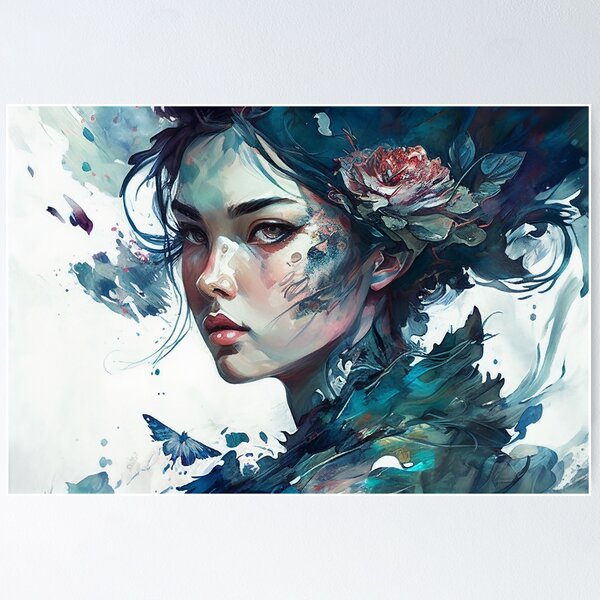This detailed piece of artwork portrays a central figure of an Asian woman with long, dark, greenish-black hair adorned with a red rose behind her left ear. She has striking red lips and slightly pink-toned skin, with a touch of blue on her left cheekbone, reminiscent of a tattoo or artistic design. Her expressive eyes and finely shaped black eyebrows seem to gaze into what would be the camera. Surrounding her head and shoulders are butterflies and leaves, adding a whimsical feel to the image. She is dressed in green and blue clothing, which complements the greenish tones in her hair and the primary colors of blue and green that dominate the image. The setting is on a background of white or light gray canvas, providing a crisp contrast to her vivid attire and the vibrant colors of the artwork. The style suggests a digital rendition with an oil painting effect, meticulously designed to capture both realism and artistic flair.